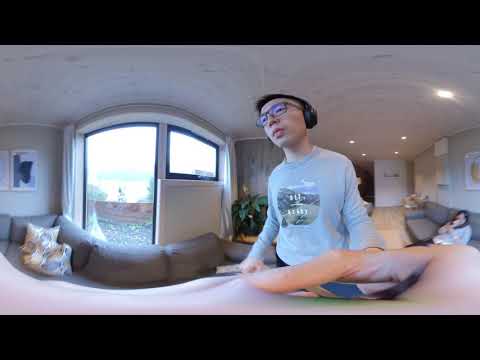The image shows an indoor scene featuring a blurred selfie of a young man of Asian descent. He is wearing headphones, glasses, and a gray or pale blue sweatshirt with some indistinguishable lettering on the front. The man is holding a phone or camera in his hand, which is visible at the bottom of the frame. The interior setting includes a tan or light brown multi-cushion sofa placed in front of large double windows with arched tops, casting natural daylight onto the scene. Through the windows, a body of water and greenery are faintly visible, suggesting a lakeside view, and hinting at an outdoor patio. Behind the young man, on the right side of the photo, a woman with long dark hair, wearing glasses, a blue top, and dark slacks, is seen sitting and possibly eating discreetly. The room has white walls, a white ceiling with recessed lighting, contributing to a bright and cozy atmosphere. The blurred nature of the photo adds to its candidness, with details like the hand appearing in the foreground, creating an intimate yet obscured snapshot of a comfortable, lived-in space.